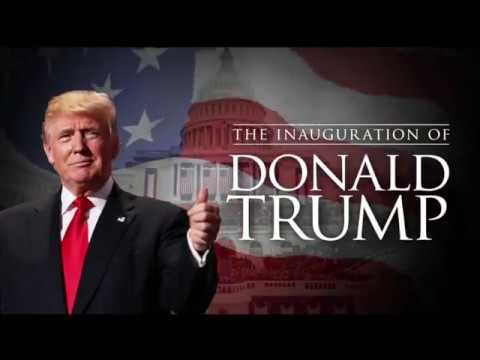This political advertisement features an image of Donald Trump on the left side, shown from the waist up. His right hand is giving a thumbs-up gesture, although it is slightly cropped by the edge of the image. Trump is wearing a black business coat adorned with an American flag lapel pin, a white collared button-up shirt, and a red tie. His thin, orange-dyed hair contrasts with his slight smile. The background combines a transparent, waving American flag and the United States Capitol building, giving a sense of patriotic fervor. The flag's blue section with white stars is in the upper left corner, though only a few stars are visible. The image also includes bold white text on the right side that reads, "The Inauguration of Donald Trump." This text, along with Trump's poised position and the iconic imagery in the background, suggests a celebratory and momentous occasion. The overall color palette includes shades of black, blue, white, yellow, red, and a nuanced interplay of transparency, creating a visually impactful scene that appears to be a screenshot from a television program or digital advertisement.